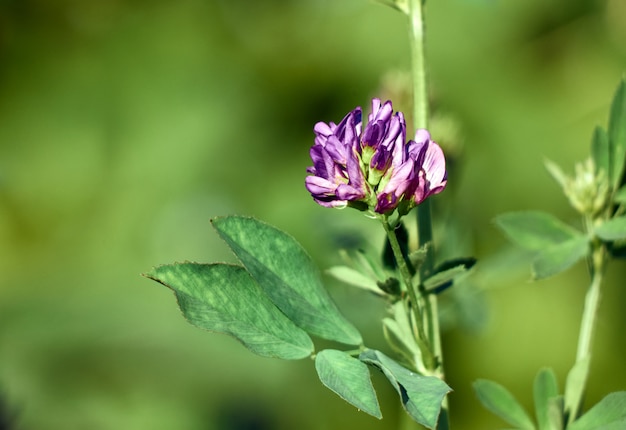This macro photograph captures a striking purple flower set against a dramatically blurred green background, allowing the vibrant blossom to be the sole focal point. The flower's long, slender green stem supports its striking array of petals, which transition in color from light to dark purple, radiating outward from a green center where the flower initially budded. A nearby offshoot features another stem that hints at a future bloom, with its bud yet to open. Complementing the composition, semi-green leaves protrude from the sides of the stems, adding depth and texture. The soft blur of the background, tinged in various shades of green, further accentuates the vivid purple flower, while hints of other out-of-focus floral elements linger subtly in the distance, unifying the natural harmony of the scene.